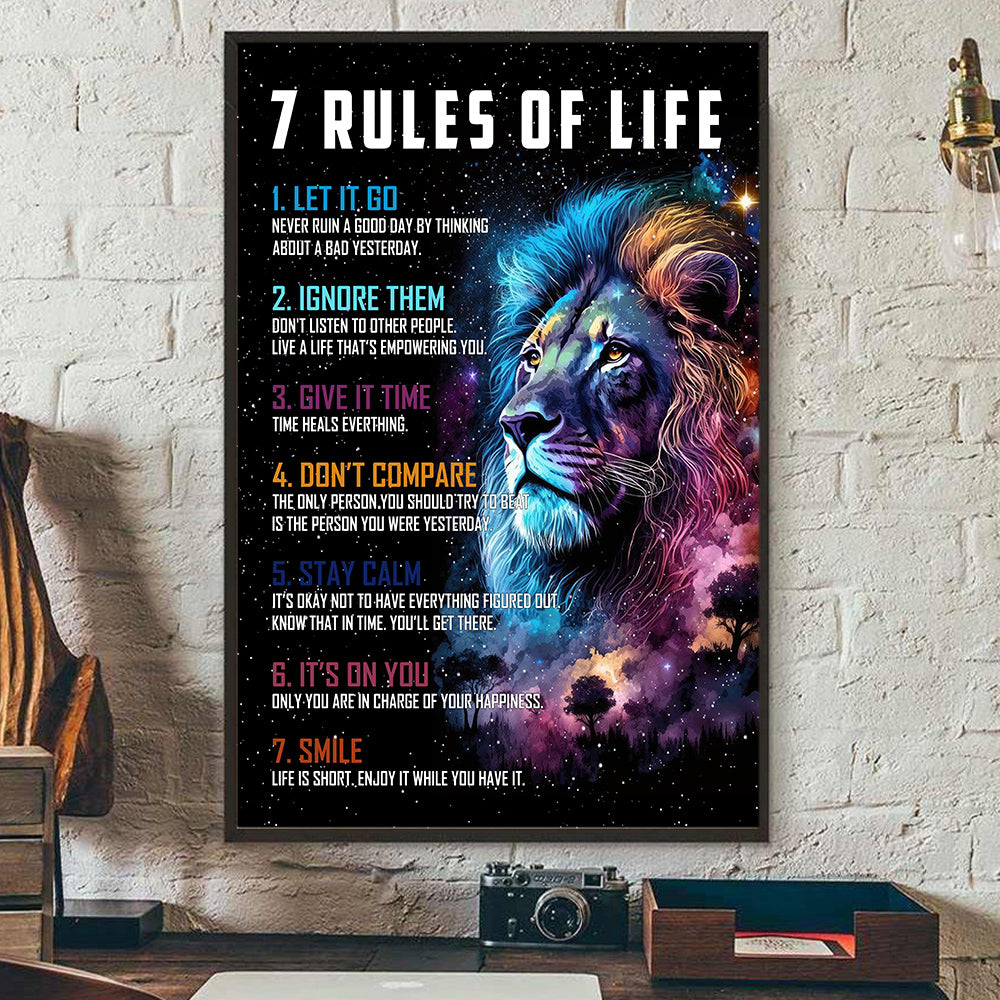The image depicts an inspirational poster hanging on a white brick wall in an office setting. The poster, vertically oriented, features a space theme with a black background adorned with stars and colorful gaseous clouds. At the center, a realistically drawn male lion is prominent, rendered in vibrant shades of blue, pink, and orange, blending into the celestial backdrop. The lion's face is primarily shown in profile, with an electric blue hue on the left and warm oranges and pinks on the right. Above the lion's head, the poster is titled "Seven Rules of Life," and below, it lists the rules: "Let it go, Ignore them, Give it time, Don't compare, Stay calm, It's on you, Smile," each with brief descriptions. Below this striking artwork, a brown wooden desk is set against the wall, holding a variety of items including a black and silver adjustable camera, a wooden outbox, a three-drawer organizer, a wooden sculpture, and what appears to be a violin on the left side. The overall scene gives a sense of a creatively inspirational workspace.